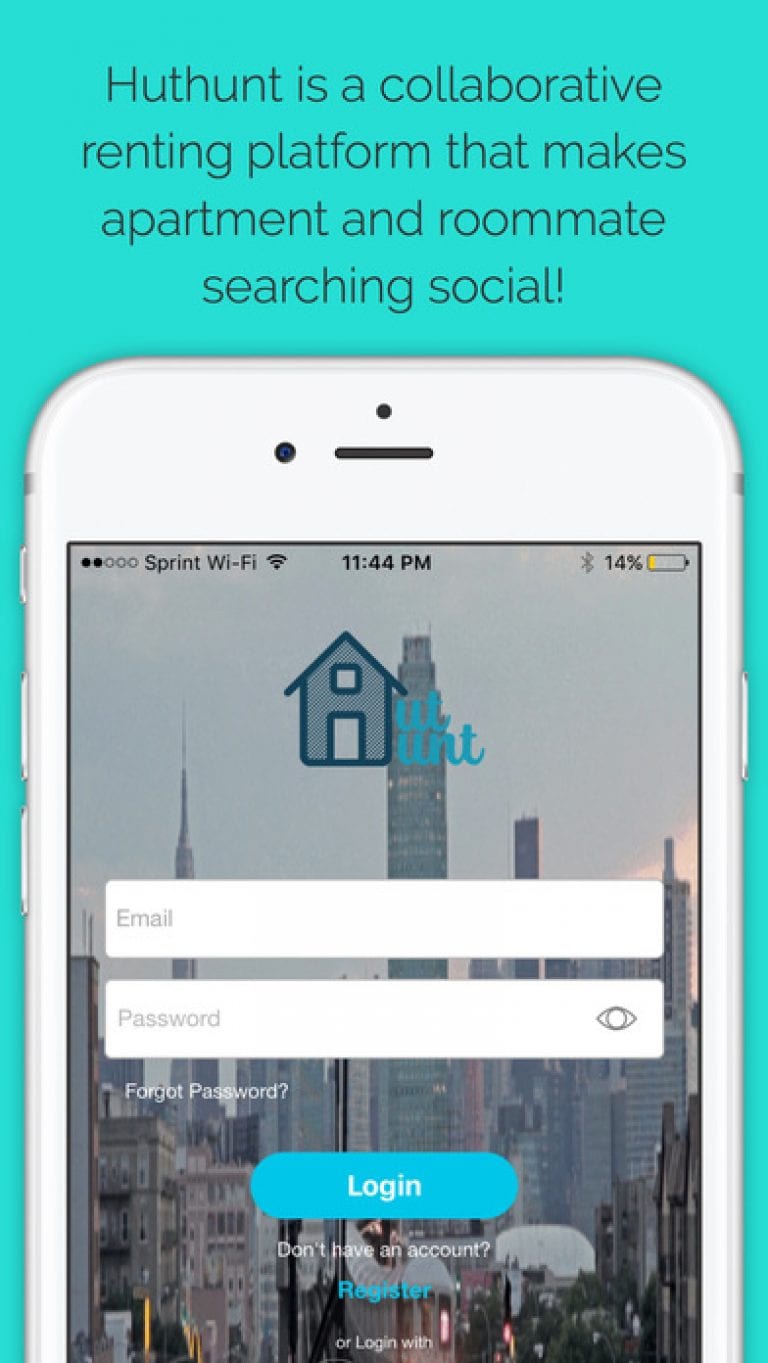This image captures a screenshot of a partially visible webpage featuring a white digital phone representation against a teal background. The screenshot reveals the top-left and right sides of the phone, but the bottom portion is cut off, suggesting there is more to the page that is not displayed.

At the top of the image, large text reads "Hut Hunt," a collaborative renting platform designed to make apartment and roommate searching a social experience, emphasized with an exclamation point. The phone’s screen shows three buttons on the left-hand side and one button on the right. The status bar at the top of the digital phone displays two out of five black dots for signal strength, the time as 11:44, and a battery charge of 14%.

Beneath the status bar is the Hut Hunt logo, where the "H" is creatively designed to resemble a house. The form on the phone’s display contains input fields labeled "Email" and "Password," followed by a "Forget Password" link. Below these fields is a teal "Login" button. Further down, the screenshot includes prompts for users who don't have an account, offering a blue "Register" button or an alternative "Login with" option.

Overall, the screenshot provides a glimpse into the user interface of the Hut Hunt platform, emphasizing its user-friendly design and social connectivity features.